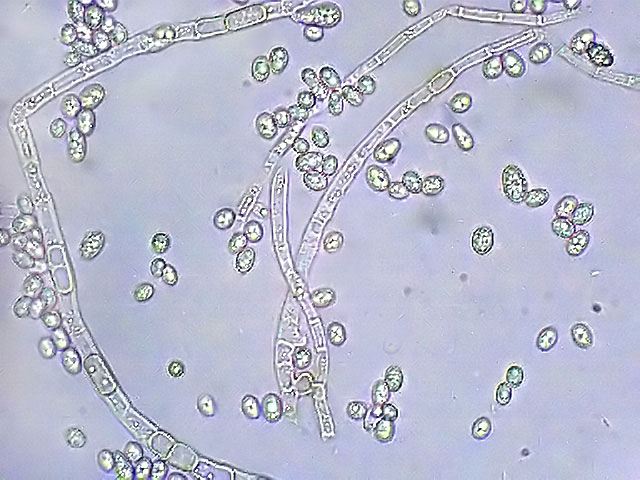This micrograph reveals a fascinating array of microscopic organisms or cellular structures against a varied background. The scene is dominated by clear, elongated shapes resembling amoebas or possibly elongated cells, alongside circular or oval forms that might be cellular components or individual cells. The primary background color shifts between shades of blue and light blue, interspersed with light gray and accented with subtle speckles. Some of the clear forms exhibit faint hints of light green, adding a delicate touch of color. These organisms or structures are scattered throughout the image, creating a complex and intricate biological tableau.